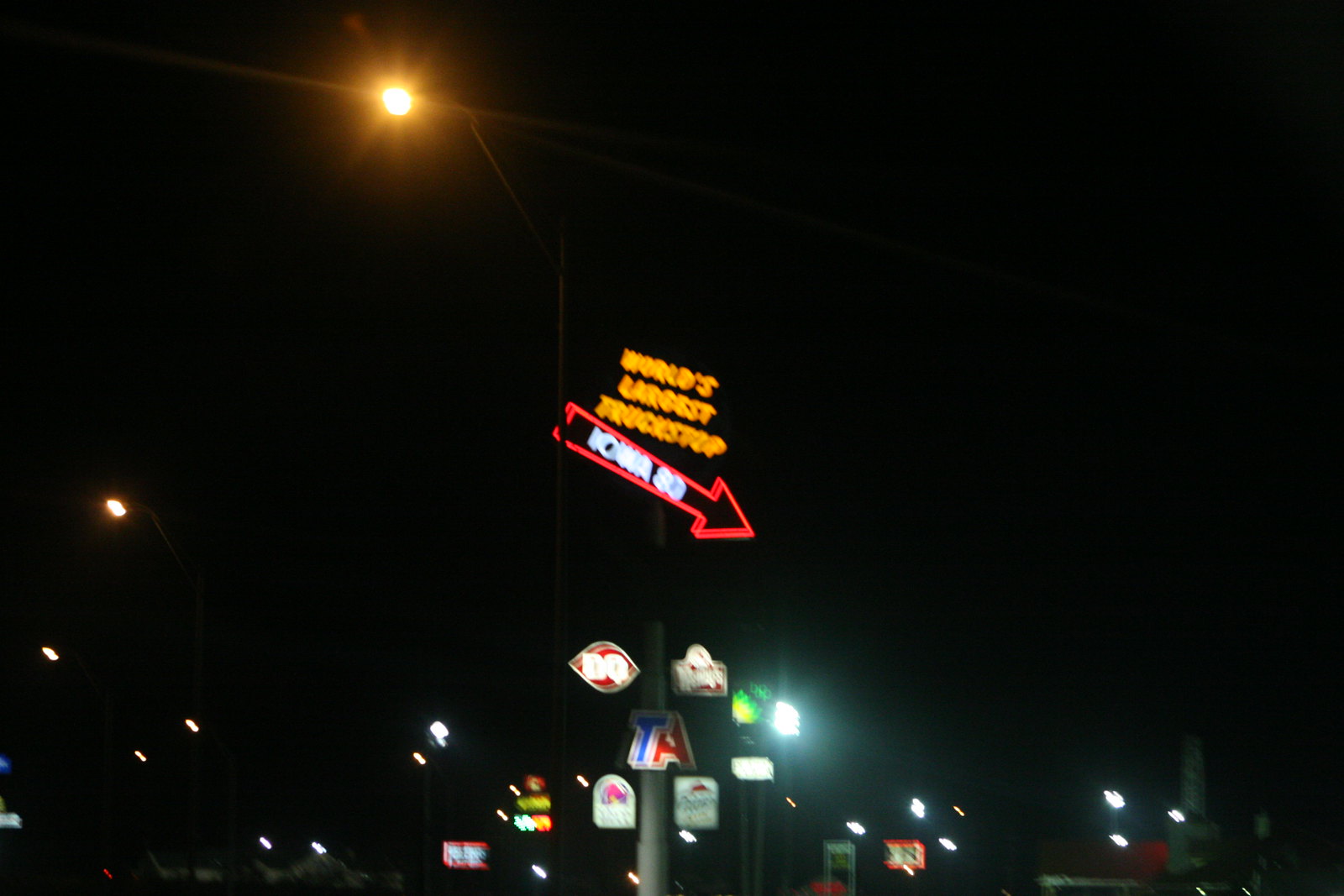This nighttime urban scene captures an upward view of a collection of illuminated signs. Dominating the image is a large sign that reads "World's Largest Truck Stop" in vivid orange text. Below this is a red outlined arrow pointing towards the bottom right corner, featuring the text "Iowa 80" in white. Beneath this prominent sign, there's a cluster of additional signs: a Dairy Queen (DQ) sign, a Wendy's sign, and another sign displaying "T" in blue and "A" in red, indicating a TA travel center. To the left of these, a Taco Bell sign is visible. Further in the background, more signs can be seen, albeit slightly blurred. The sky is a deep black, typical of nighttime, accented by an orange beam of light and several orbs of light on the lower left portion, possibly from streetlights or passing vehicles, adding depth and ambiance to the scene.